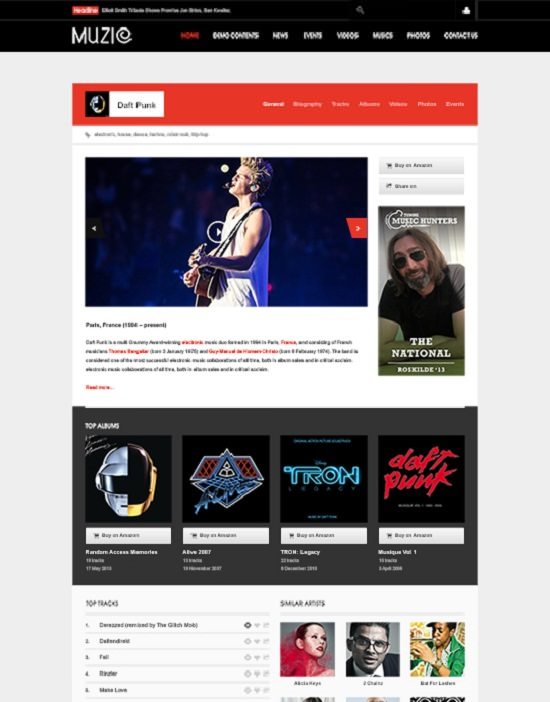This is a detailed screenshot of a website, primarily focused on a music theme. 

The webpage has a vertical orientation, being taller than wide. At the very top, there's a narrow black banner with some small, unreadable text positioned at the top left.

Below this, still within the black banner, the word "MUZIC" appears prominently, with the "C" stylized in a unique, artistic manner that makes it almost unrecognizable as a "C." 

To the right of "MUZIC," there are eight navigational sections arranged horizontally. The first section stands out in red, while the remaining seven are in white, though the text is too small to decipher.

Beneath the black banner is a solid gray box, spanning the width of the page. At the top of this gray box is a smaller red banner. On the left side of this red banner, it says "Daft Punk," accompanied by a small icon. Adjacent to this, there are multiple tabs for further navigation or selection, but these tabs are also too small to read clearly.

Directly under the red banner, there's a picture of a single white man playing a guitar. This image serves as a clickable preview or play button for a video. Below the image, there's some text which is, again, too small to read.

To the right of the guitar-playing man image, there's an advertisement featuring a long-haired man with glasses and a beard, labeled "The National."

Below this main content area, a solid black banner stretches across the width of the page. It contains four clickable items, each accompanied by images—a helmet-like object, an emblem, the Tron movie symbol, and an image representing Daft Punk. Each image has a white box beneath it with some unreadable text.

At the very bottom of the page, on the left side, there's a section listing several music tracks, although the text is too small to be read. On the right side, there are three pictures of faces, possibly music stars, indicating a "similar apps" section.